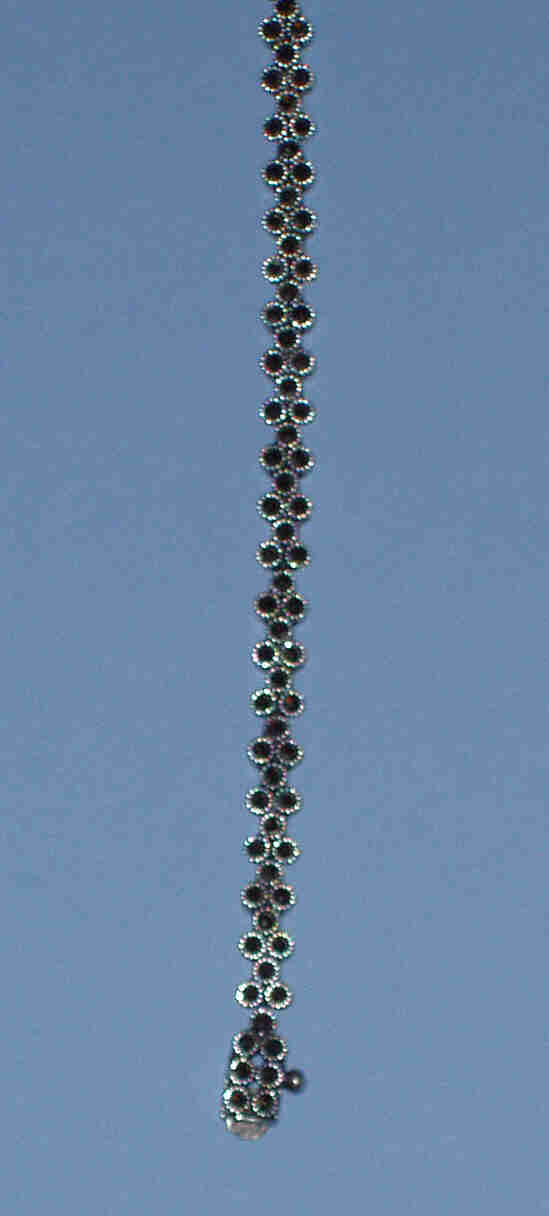The photograph features a delicate piece of jewelry laid out on a medium blue background. The intricate design comprises a series of tiny flowers, each with silver petals and a black center. Arranged in a visually appealing pattern, the flowers alternate between single and paired formations, which gives the impression of larger blooms. The detailed craftsmanship makes this bracelet appear almost as part of a larger collection of fine jewelry. A sophisticated clasp is visible on one end, while the photo cuts off the other end. The overall composition of the bracelet suggests it's ideal for complementing an evening dress. Despite varying interpretations, the key elements—delicate silver and black flowers set against a blue-gray backdrop—remain prominent in portraying this exquisite item.